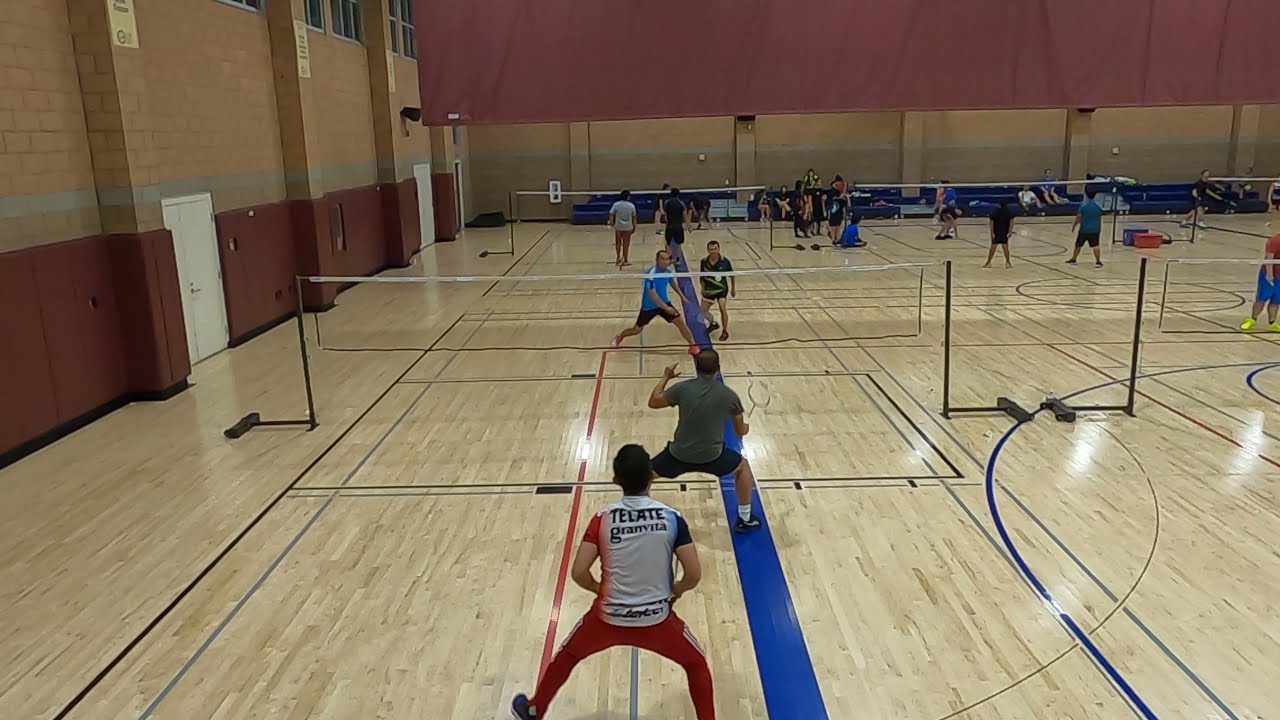This horizontally aligned rectangular photograph captures an energetic scene inside a large indoor gymnasium with beige, wood-grain floors featuring blue, black, gray, and red court lines. The walls are a mix of tan and reddish-brown stone, with sections painted maroon near the bottom. Several badminton games are in progress, with numerous courts set up, indicating a bustling atmosphere with approximately 10 to 15 people involved in different matches. 

In the foreground, a man wearing red Adidas athletic pants and a distinct white, red, and blue jersey labeled "Tilati Gran Vita" is prominently positioned, poised for action. The jersey features a unique design with a navy right sleeve and a red left sleeve. In front of him stands an opponent, dressed in a gray short-sleeve shirt and black shorts, gripping his racket in anticipation. Across the net, two more competitors are present— one in a blue shirt, just having hit the shuttlecock, and another in black, ready for the next move. 

The background reveals additional games, with multiple badminton nets arranged closely together, indicating at least three courts side by side and more extending into the distance. The bright light casts a shine on the polished floor, accentuating the enthusiastic atmosphere within this well-used gym.